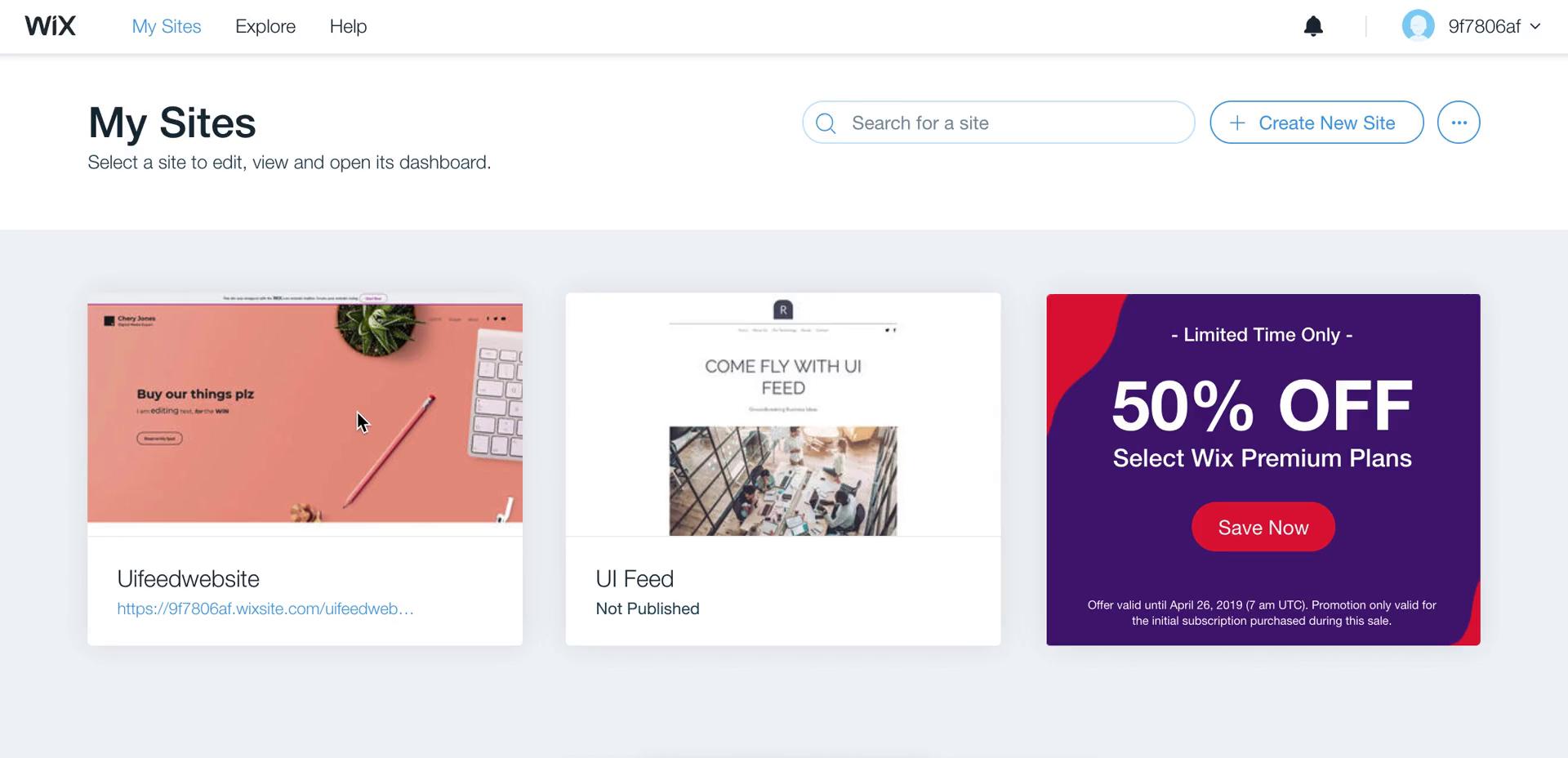**Descriptive Caption:**

"Screenshot of the Wix dashboard interface showcasing the MySite management area. At the top, a white navigation bar includes options for Wix, MySite, Explore, and Help, along with a notification bell icon and a generic profile picture. A unique identifier '9F7806AF' is displayed beneath these elements. Below, a gray horizontal line separates the navigation bar from the main content area. The interface instructs users to 'Select the site to edit. View and open its dashboard.' There is a prominent search bar encouraging users to 'Search for a site' with a magnifying glass icon beside it, followed by a 'Create New Site' button.

In the central section, a circular button with an ellipsis symbolizes more options. The background here is gray. On the left, a thumbnail image of a pink surface with a pencil and keyboard reads 'Buy Our Things Please' with a caption 'UI Feed Website' underneath, flanked by a blue hyperlink. Adjacent in the middle, another thumbnail offers an aerial view of an office with the directive 'Comply with UI Feed.' The rightmost thumbnail features a dark purple background announcing 'Limited Time Only. 50% Off. Select which premium plan,' accompanied by a bold red 'Save Now' button."